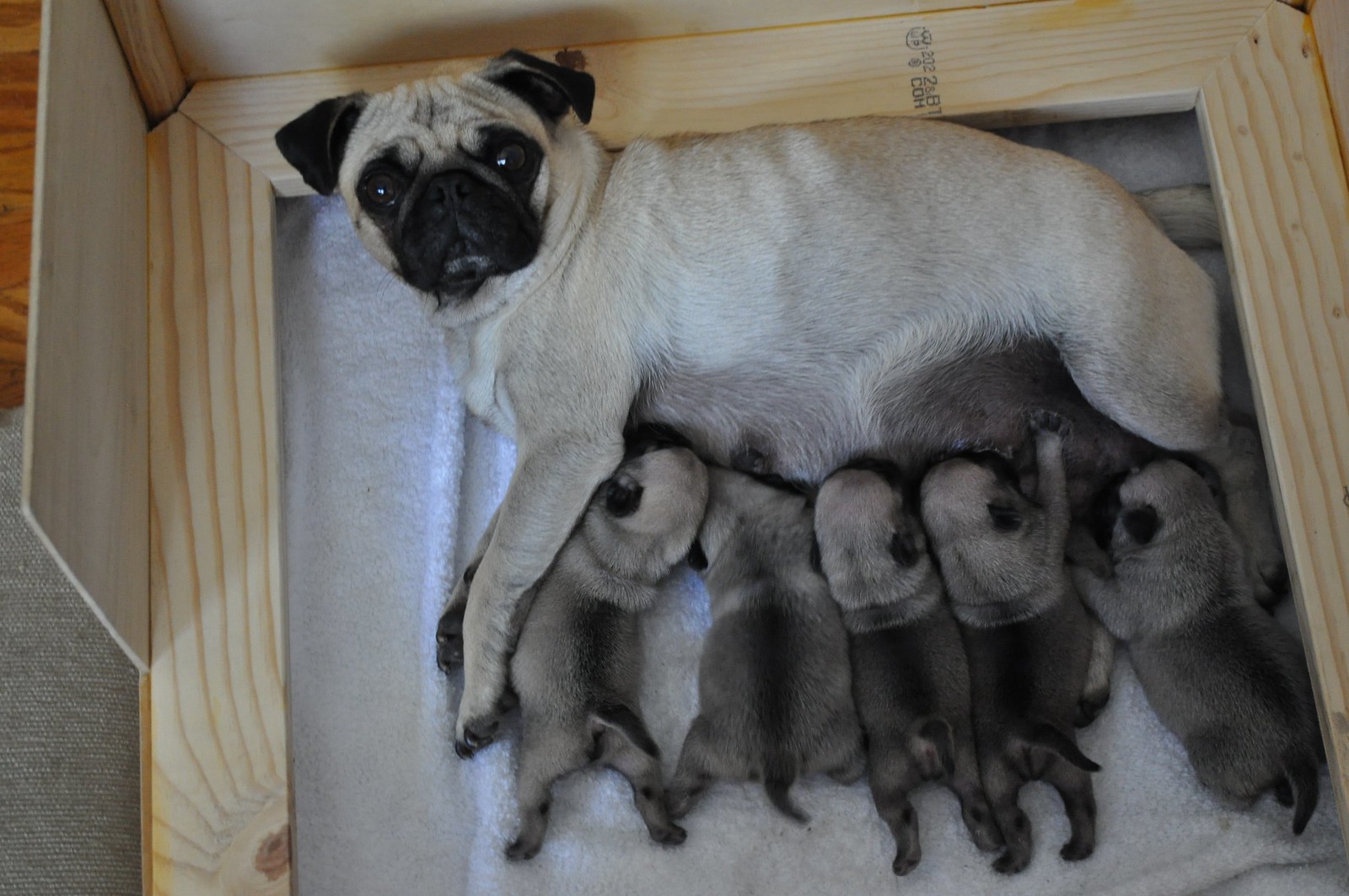This color photograph captures a heartwarming scene of a female pug nursing her five puppies. The rectangular, horizontal image offers a top-down view into a hand-built wooden nesting box made of two-by-fours and thin plywood, lined with a blanket and towel for comfort. The pug mother lies on her right side, gazing up at the camera with her bright eyes, her black snout, ears, and eye area contrasting against her light gray or grayish-brown fur. The nursing puppies, darker in color with medium gray around their heads and darker gray to black bodies, are positioned from beneath her front legs to near her hind legs. The mother's front left paw rests over one of the puppies, while her curled tail peeks out from under the edge of the wood. This charming snapshot captures the tender bond between the mother pug and her newborns in their cozy, homemade nesting crate.